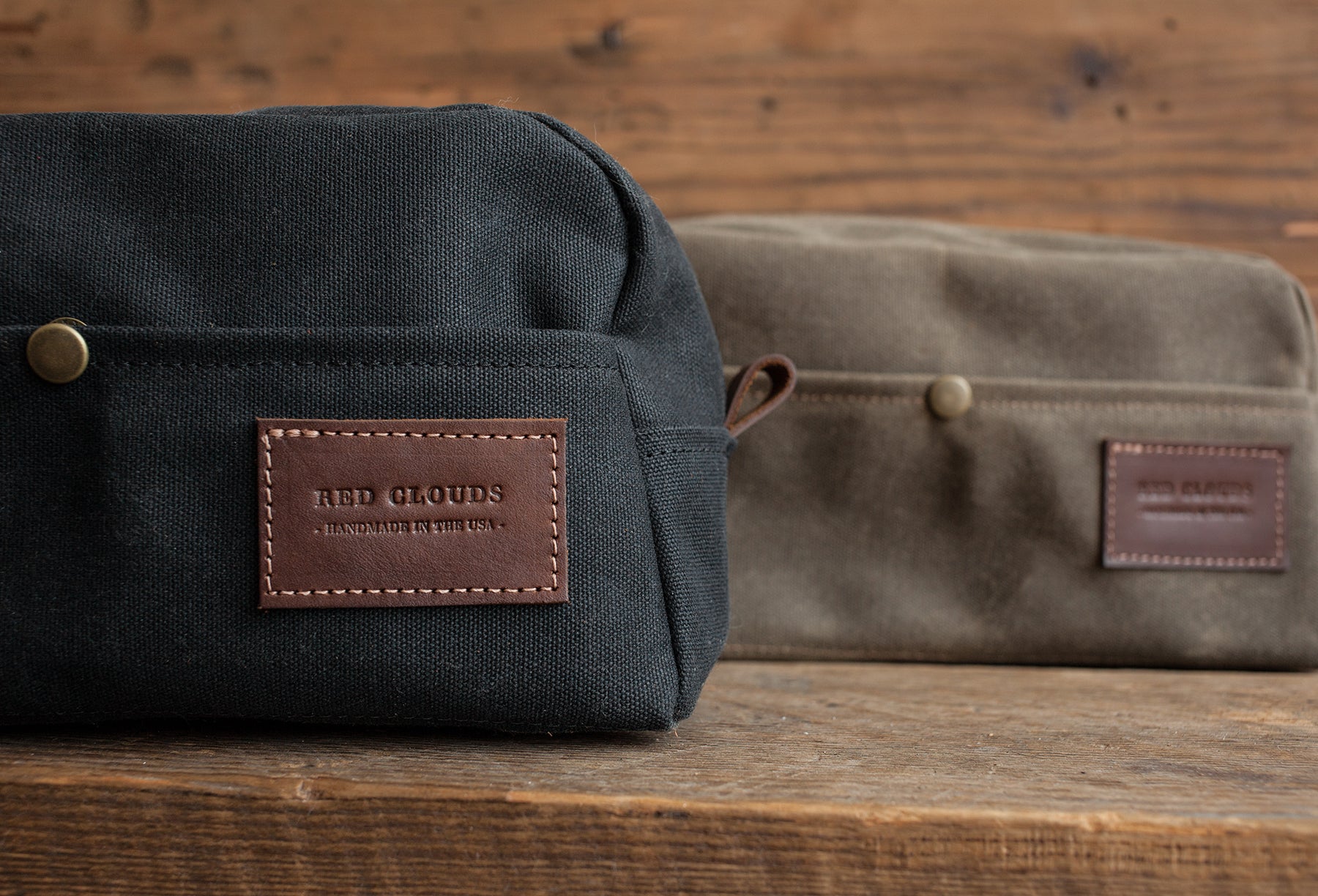The image features a wooden desk with two canvas bags placed on it. The bag on the left is primarily black charcoal gray, featuring a prominent brass button in the center. It is adorned with a brown leather patch with visible white stitching, which bears the text, “Red Clouds, Handmade in the USA.” The bag on the right is a blue hue with a brownish tint and has a similar leather patch with text, as well as its own central button. Behind the bags, a wooden board can be seen serving as a backdrop. The detailed craftsmanship of the leather patches and the textile quality of the canvas bags stand out, highlighting their handmade origin.